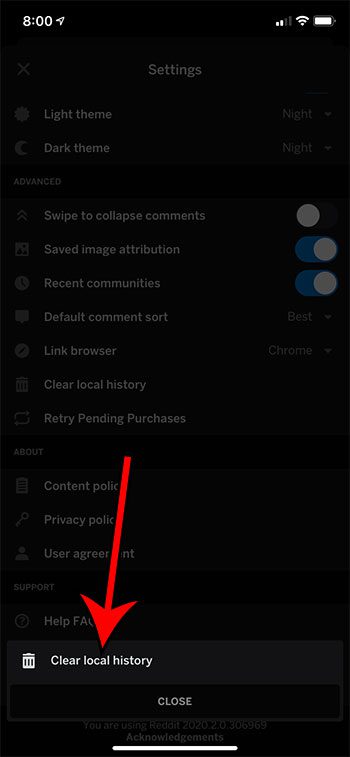The screenshot captures a phone screen displaying various settings options against a stark background transitioning from black at the top to white towards the middle. The top-left corner showcases the current time "8:00" in white, set against a black background. Adjacent to the time, a white arrow icon points to the right, indicating further navigation options.

The signal reception is illustrated by four bars, two of which are white, signaling moderate reception strength. Complementing this, the Wi-Fi icon displays fully white bars, indicating a strong and stable connection. The battery icon, predominantly white and nearly full, suggests about 90% battery life remaining.

On the left side of the screen is a gray "X" icon, presumably to exit the current settings view. Below that, in grayish-white text, is the word "Settings." This is followed by text options indicating "Light Theme" and "Dark Theme," the latter accompanied by a crescent moon icon.

Further settings include an "Advanced" section, followed by a toggle option reading "Swipe to collapse comments" with a white circle toggle on the right side. Another option, "Save image attribution," is accompanied by a white and blue oval interface element.

Beneath these options, more settings are listed: "Recent communities," "Default comment sort (Best)," and "Link browser (Chrome)." Additional options include "Clear local history" and "Retry pending purchases," followed by another section headed by "Content," partially obscured by a big red arrow. This arrow points downward, ending at the option "Clear local history" highlighted in white text.

The red arrow truncates the visibility of some options such as "Content," "Privacy," and "User Agreement," partially obstructing the text but directing the user's attention towards the "Clear local history" option at the bottom.